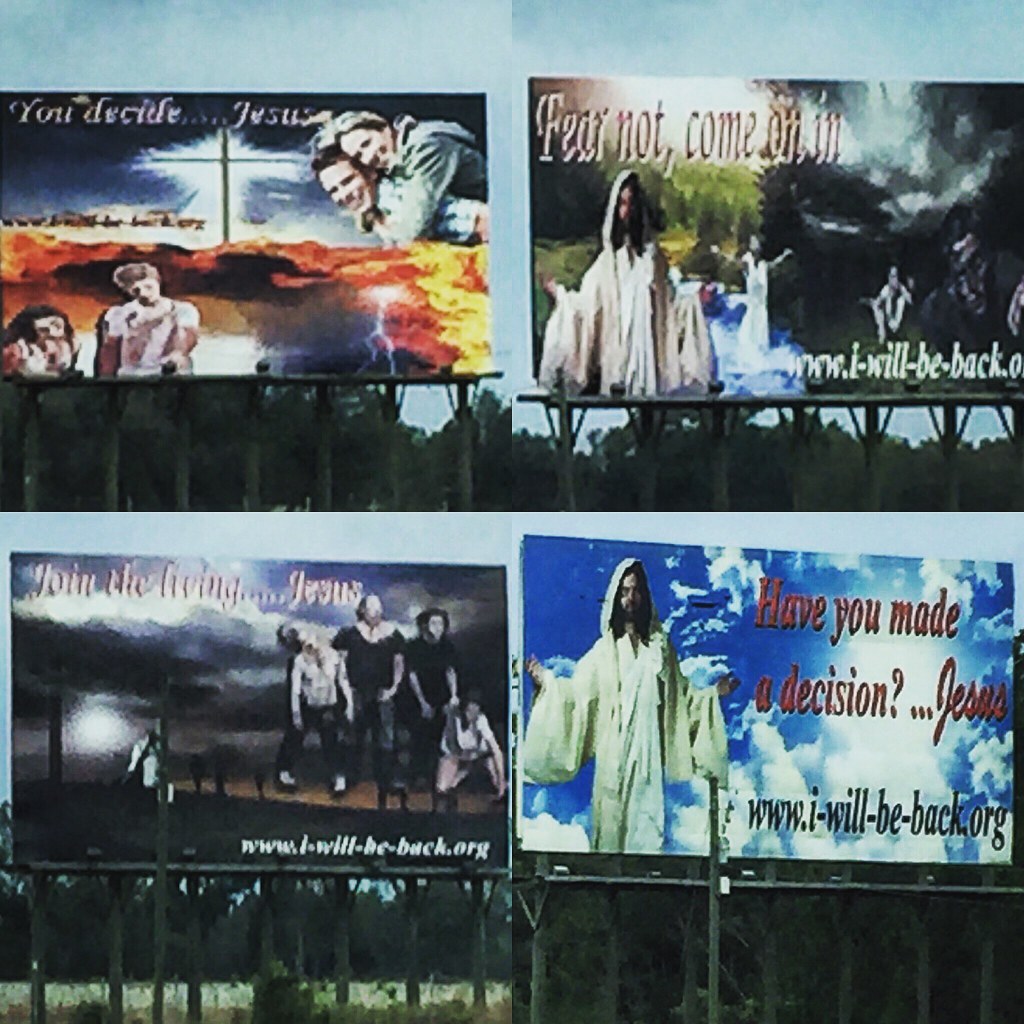This photograph is a collage of four grainy religious billboards, mounted on dark green posts, standing about 10 feet off the ground along a rural roadway with low-level trees behind. The upper left billboard, set against a yellow and orange mountain range with glowing white rays behind a cross, features a woman holding onto a man’s back and reads, "You Decide, Jesus." Below, a woman and a girl are visible amidst a fiery scene. In the upper right, the billboard displays Jesus in a white robe with arms outstretched and reads, "Fear Not, Come On In," accompanied by a woman standing in water and another sitting on the ground; it also includes the URL, "www.iwillcomeback.com." The lower left billboard, set beneath black and white clouds, reads, "Join the Living, Jesus," and features four people who resemble zombies with the URL "www.iwillbeback.org." The lower right billboard shows Jesus in a white robe against a blue sky with white clouds, reading, "Have You Made a Decision? Jesus," and also includes the URL "www.iwillbeback.org." All four images are positioned above what seems to be a gate with trees visible in the background.